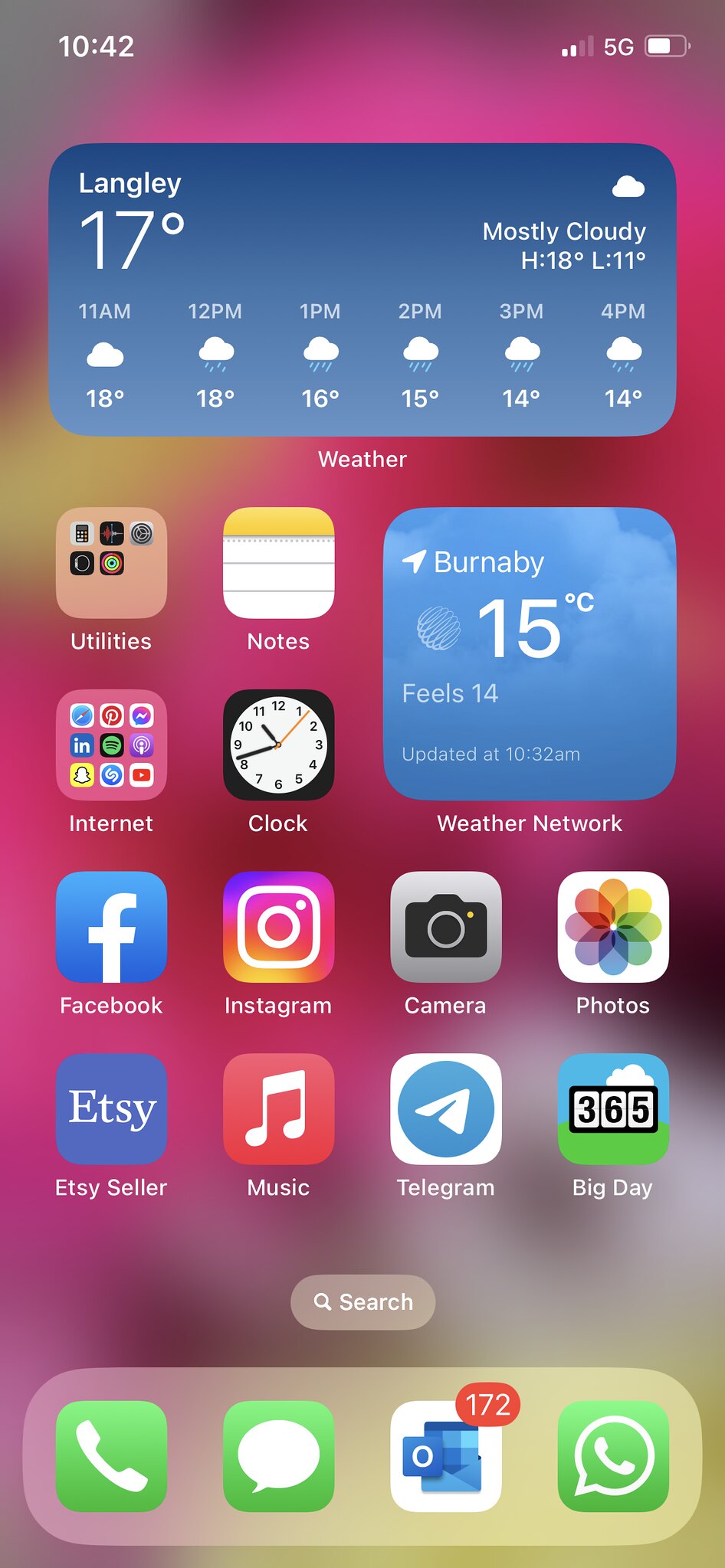This is a detailed screenshot of a smartphone, possibly an iPhone or an Android device. The background features a predominantly pink hue with subtle accents of yellow and white. At the top of the screen, various status indicators are visible, including the time, battery life percentage, and Wi-Fi signal strength. The location is shown as "Langley," with a current temperature of 17°C, described as mostly cloudy. The forecast includes a high of 18°C and a low of 11°C.

Below this information, several app icons are neatly arranged. The apps include categories labeled as Utilities, Notes, Internet, Clock, Weather Network, Facebook, Instagram, Camera, Photos, Big Day, Telegram, Music, and Etsy Seller. Additionally, there is a search button available for quick navigation.

At the bottom row of the screen, there are four more icons: a phone for making calls, a messaging app, Outlook for emails, and another phone symbol inside a call-out icon, possibly another messaging or contact app.